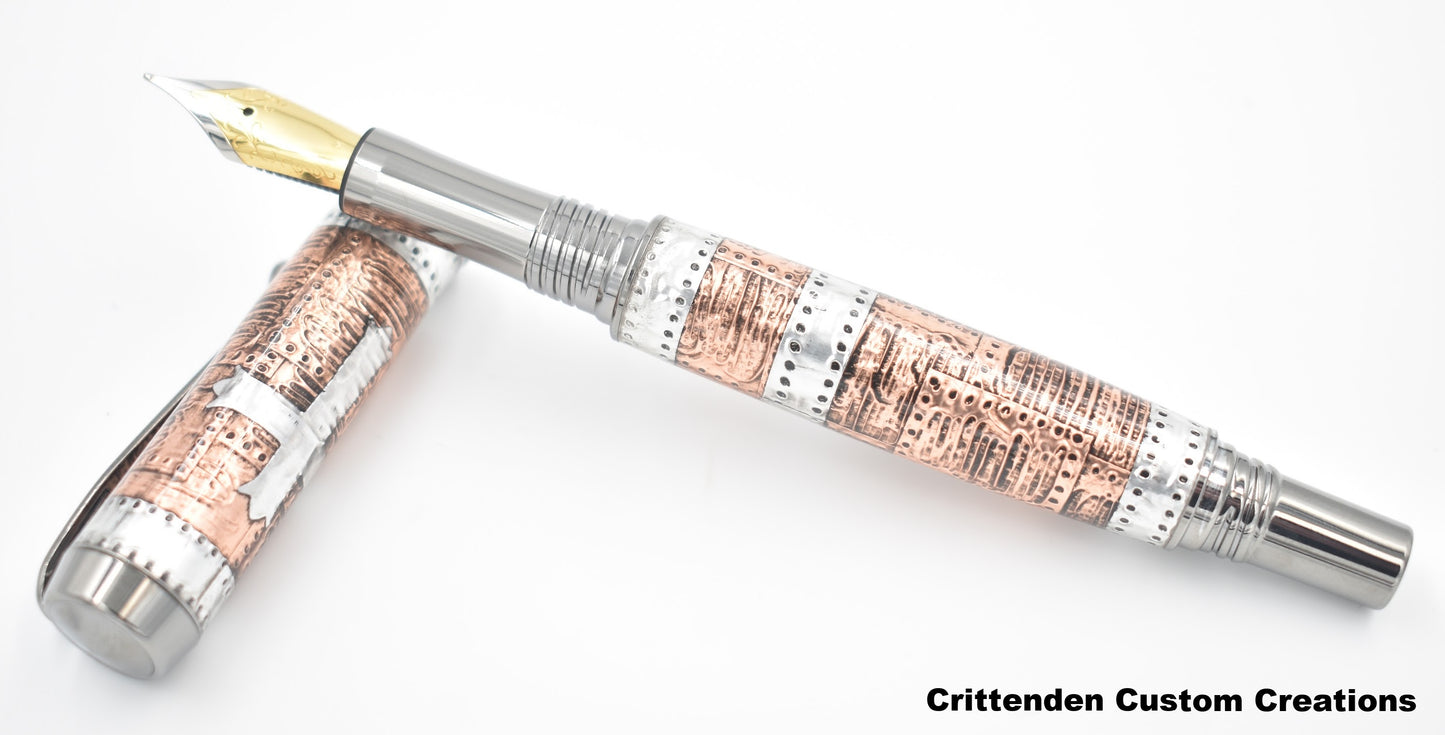The image showcases a highly stylized and fancy fountain pen resting on its screw-on cap, all set against a plain white background. The pen features a light brown, almost copper-like body, accented with steel bands and rivets that give it a flat, industrial texture. Its golden tip is trimmed with silver, and the silver chrome neck extends seamlessly into the pen's body. The rear end of the pen is flat and made of steel, mirroring the flat top of the cap. The pen cap itself bulges slightly at the end and shares the same copper-like finish as the body. Prominently displayed on the cap is a white cross with spiked ends. In the lower right corner of the image, black text reads "Crittenden Custom Creations," completing the elegant and detailed presentation of this calligraphy pen.